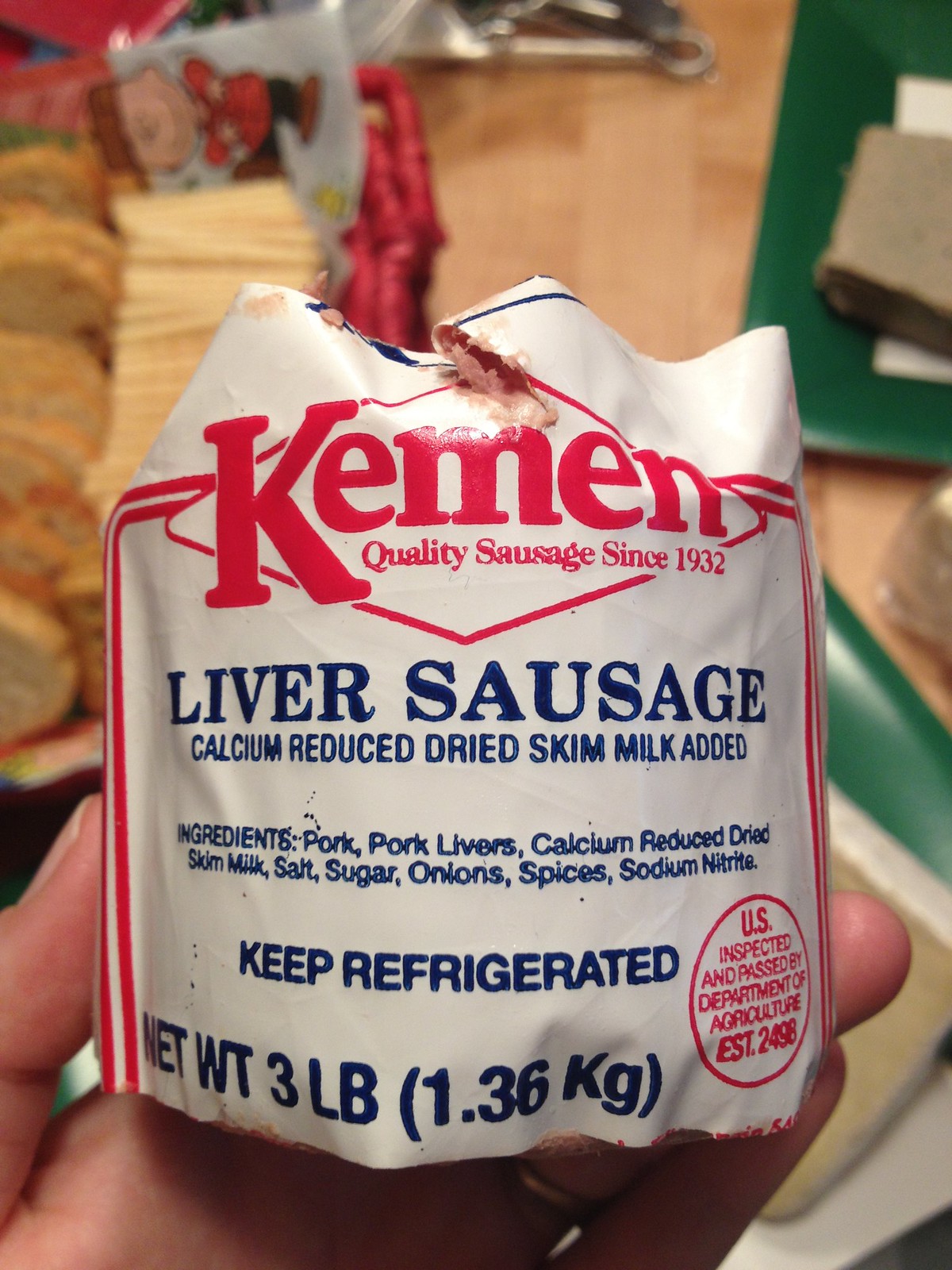The image features a packet of "Kemen Quality Sausage since 1932, Liver Sausage." The Kemen logo and the phrase "Quality Sausage since 1932" are prominently displayed in red writing against a white background, adorned with a diamond pattern around the word "Kemen." Most of the other writing on the front of the packaging is in blue, except for a small red circle containing the U.S. Department of Agriculture inspection and approval stamp.

The packaging details the product as "Liver Sausage, Calcium Reduced Dried Skim Milk Added." The list of ingredients includes pork, pork livers, calcium reduced dried skim milk, salt, sugar, onions, spices, and sodium nitrate. It also instructs to keep the product refrigerated and indicates a net weight of 3 pounds (1.36 kilograms).

In the background, there is a table with various pieces of food arranged in baskets. A human hand is holding up the packet of liver sausage, and the packet appears to be open.